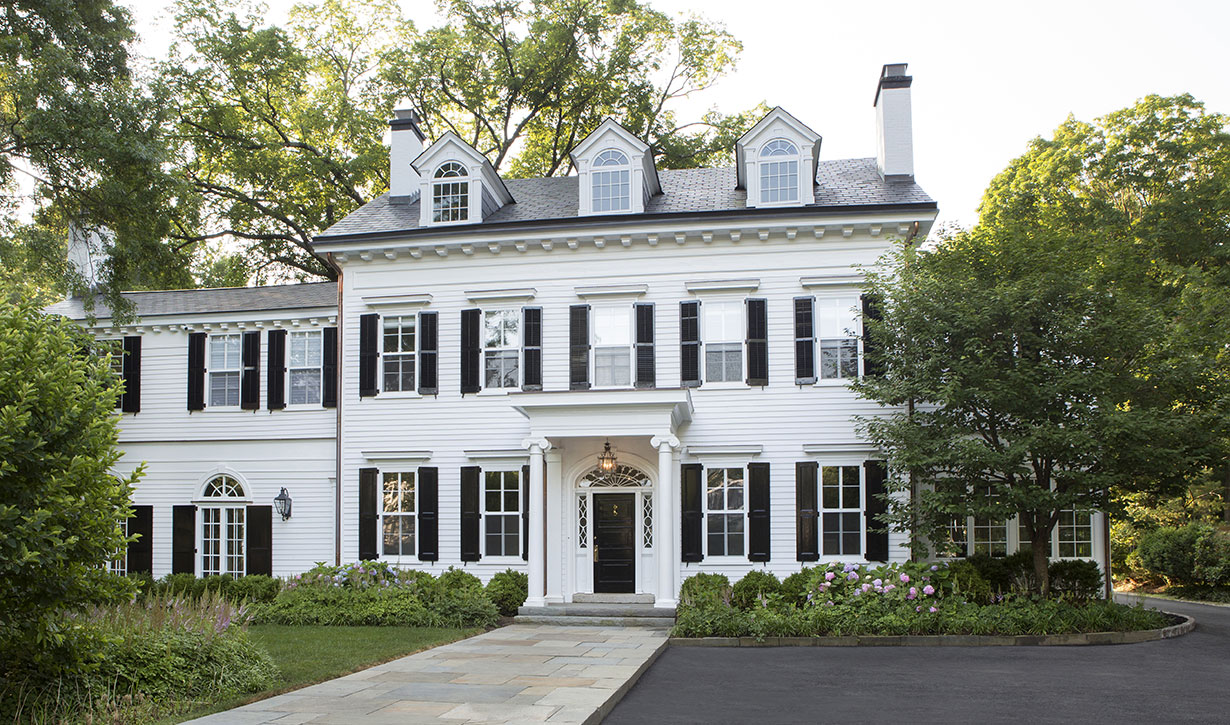This image showcases a grand, white colonial-style house, possibly a renovated plantation home, surrounded by towering green trees that offer a shaded ambiance. The house features three stories, with the top floor being an attic punctuated by three arched, triangular windows. The symmetrical façade proudly displays numerous small white windows, all adorned with black wooden shutters, except for the large windows in the day room extension on the right which remain unshuttered. There's a total of five windows across the top row and two on each side of the central entrance on the first floor. The stately black front door, centered beneath a white wooden awning supported by columns, is bordered by decorative sidelights. A walkway of interlaid light gray and brown bricks starts from the bottom left corner of the image, leading diagonally to the entrance. To the right of this path, a black paved driveway provides access. Additionally, a well-manicured garden with green bushes sprinkled with pink flowers enhances the landscape, complemented by lush lawns on either side. The house is flanked by two fireplace chimneys, and its elegant design evokes the charm of notable film settings like the home from "Father of the Bride."